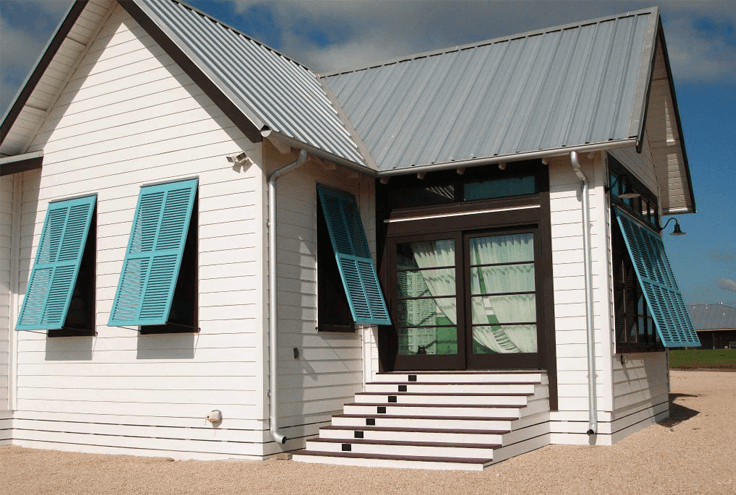This photograph depicts an isolated, small beach house prominently situated on a sandy or gravel plot, possibly near water with distant land visible. The house, characterized by its white horizontal siding, has a traditional triangle roof clad in gray steel shingles. The distinct roof features visible ridges and is equipped with a gutter and downspout system. A notable aspect is the blue paneled window shaders, all hinged at the top and propped open from the bottom, suggesting ventilation or insect prevention. 

A set of brown-topped, white-supported stairs lead up to a double door, likely a rear entrance adorned with drapes and a small overhead window. The white house is highlighted against a backdrop of a dark blue sky with patches of gray clouds, indicative of an impending rain. Despite the presence of other structures at a distance, this house stands alone, emphasized by the clear, unobstructed sandy surroundings. Overall, the house exudes a quaint, serene beachside charm enhanced by its simple, yet functional design elements.